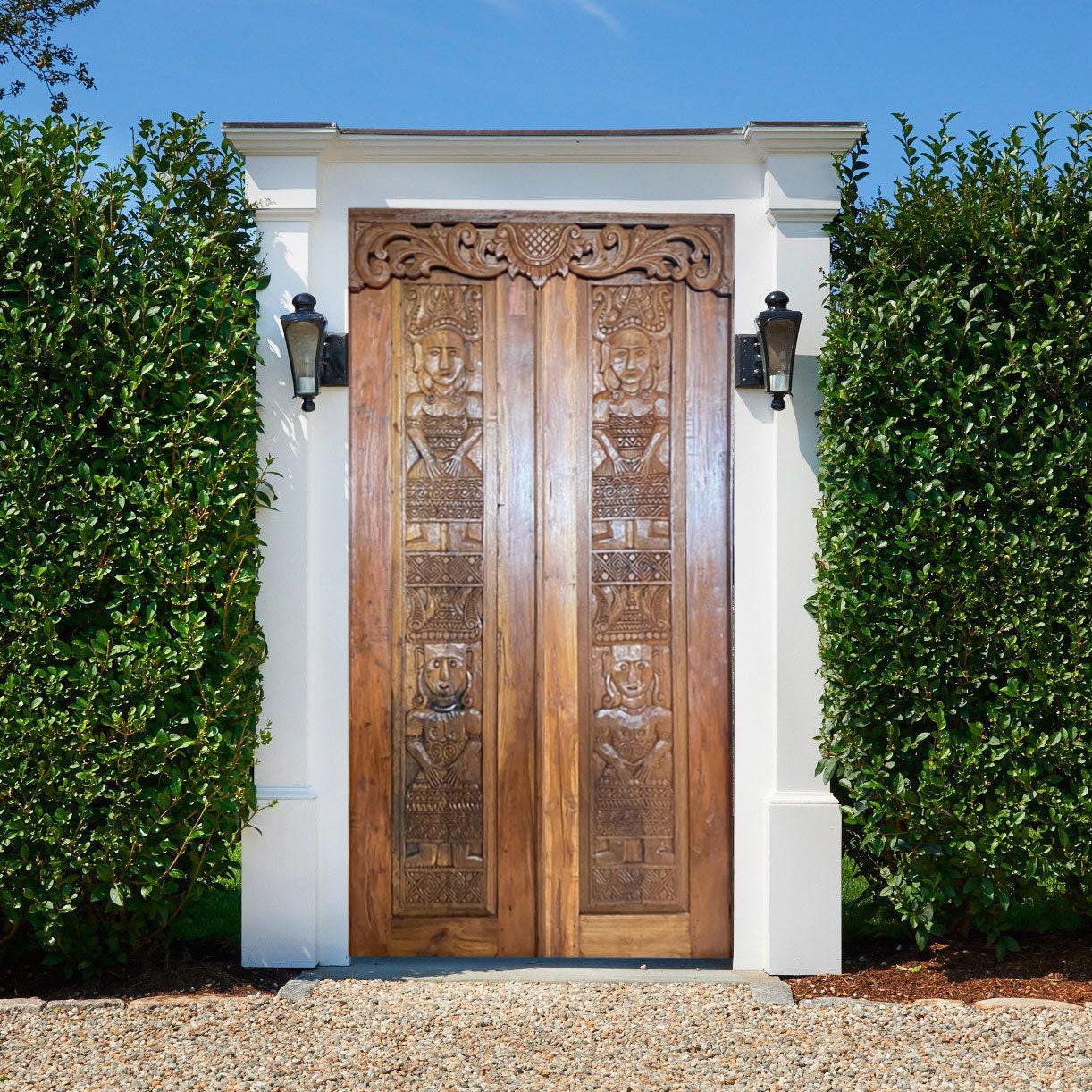The image depicts a large, intricately designed wooden door framed by a white structure. The door, rich in carvings, features what appear to be figures of tribal or native peoples, possibly of royal or religious descent, dressed in traditional tunics. On either side of the white frame are sconces, adding to the ornate detailing. Surrounding the entrance are tall, lush, dark green bushes in full bloom, likely eugenia hedges, which create a natural, enclosed setting. The pathway leading to the door is made of gravel, suggesting it could lead to a private garden, property, or even a temple, given the intricate and possibly cultural design elements.